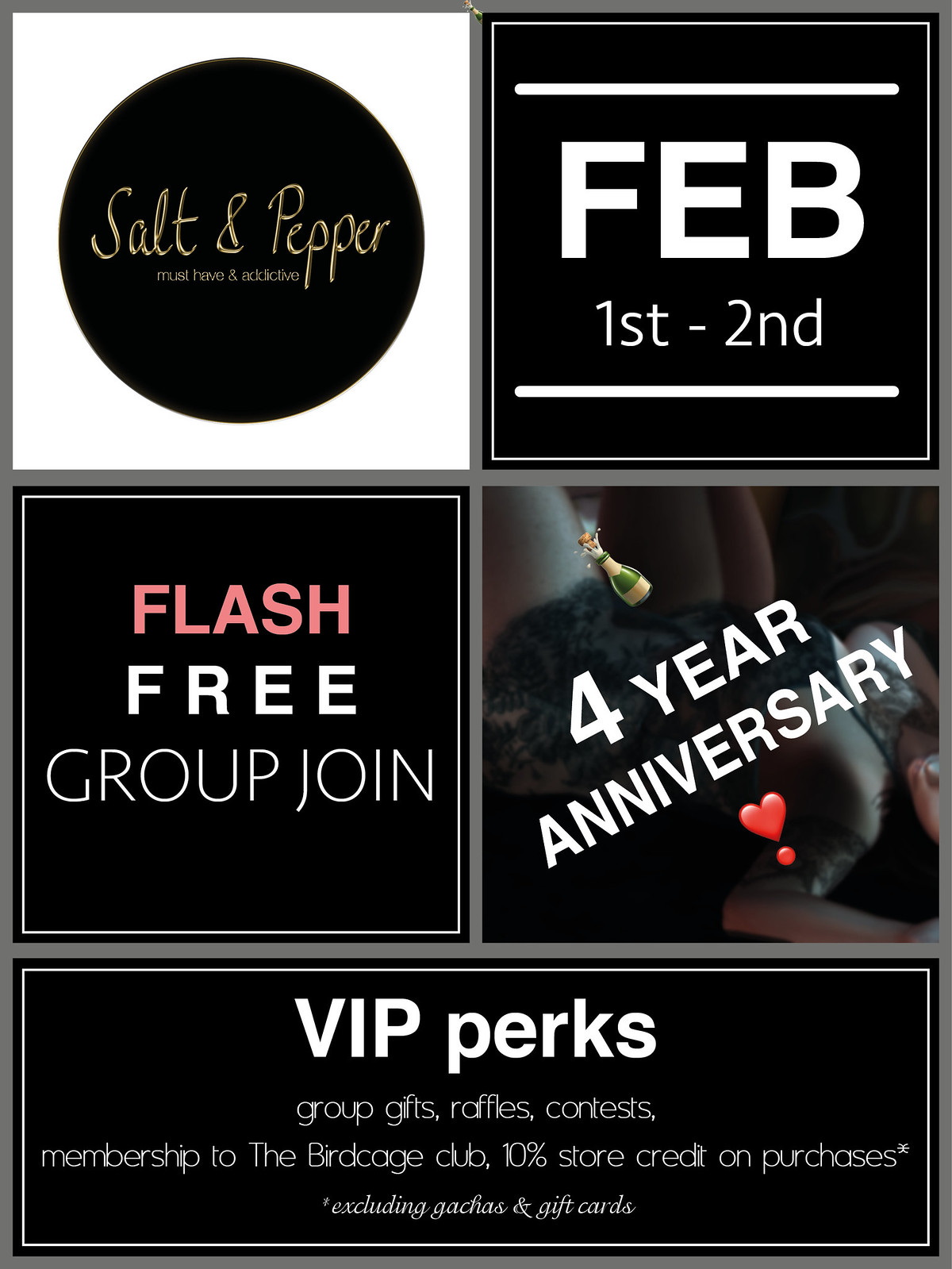This advertisement for Salt and Pepper is structured into five sections: four squares at the top and a longer rectangle at the bottom, all set against a gray background. The top left square features a black circle with the Salt and Pepper logo in yellow cursive text on a white background. To the right, the next square highlights “February 1st and 2nd” in prominent white text with thin white lines above and below it. The bottom left square reads “Flash” in pink and “Free Group Join” in white text. Adjacent to this, the right square celebrates the "Four-Year Anniversary" with white diagonal text, accompanied by a champagne bottle and heart emoji. Beneath these squares, the longer rectangular section lists “VIP perks” in bold white text and includes benefits such as group gifts, raffles, contests, membership to the Birdcage Club, and a 10% store credit on purchases, excluding gotchas and gift cards. The advertisement is primarily graphic without any photos.